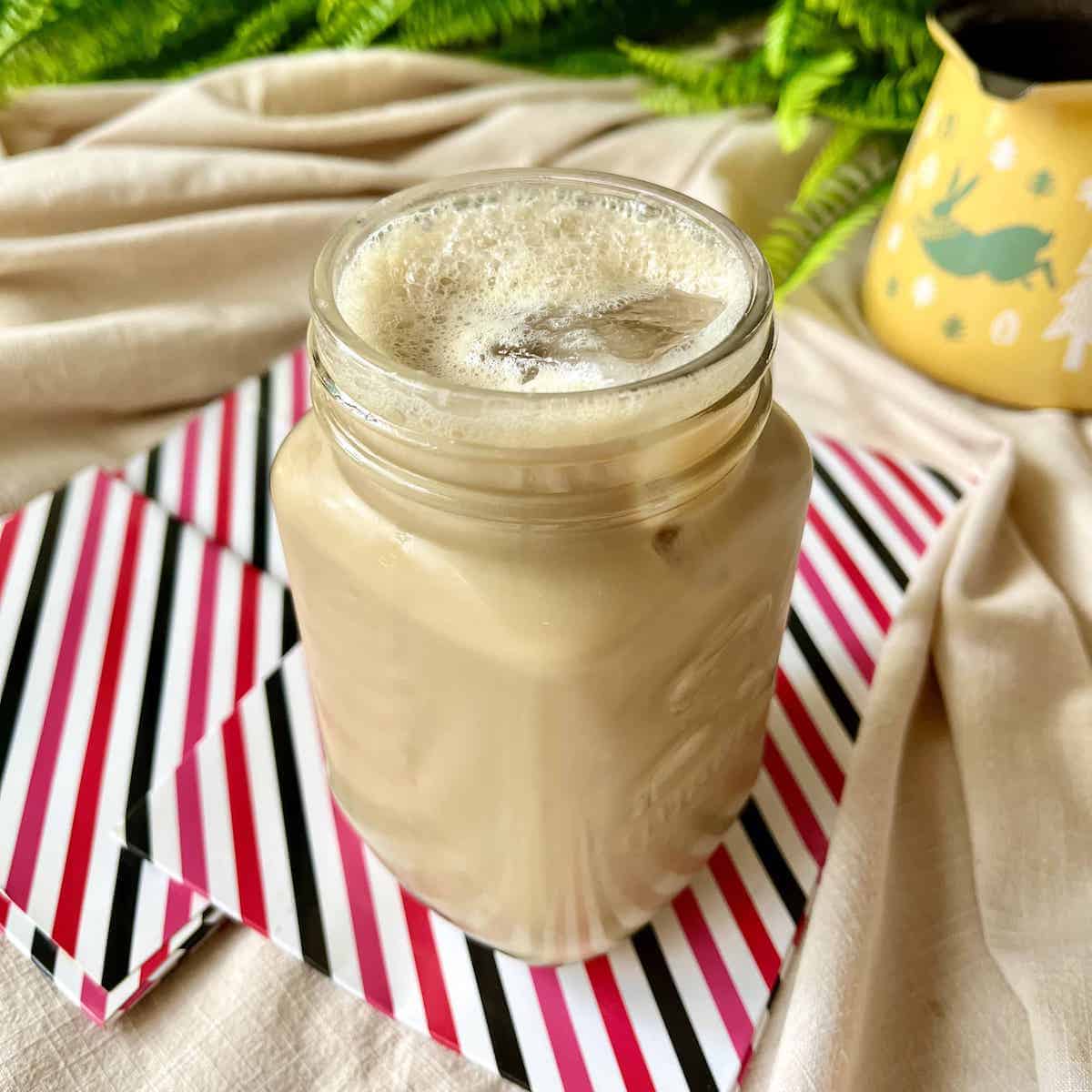This outdoor photograph captures a refreshing drink presented in a mason jar that sits on a stylish napkin with black, pink, and white stripes. The table, adorned with a white muslin tablecloth, is set in a natural, picnic-like environment, evidenced by the surrounding ferns and green leaves. The mason jar contains a brownish, creamy liquid, likely an iced coffee or horchata, with visible ice cubes and a foamy top, evoking a sense of cool delight perfect for a summer day. Also on the table is a charming yellow pot featuring a painted bunny, adding a whimsical touch. This beautifully composed image, likely intended for social media, emphasizes a relaxed, summery vibe through its rustic and colorful elements.